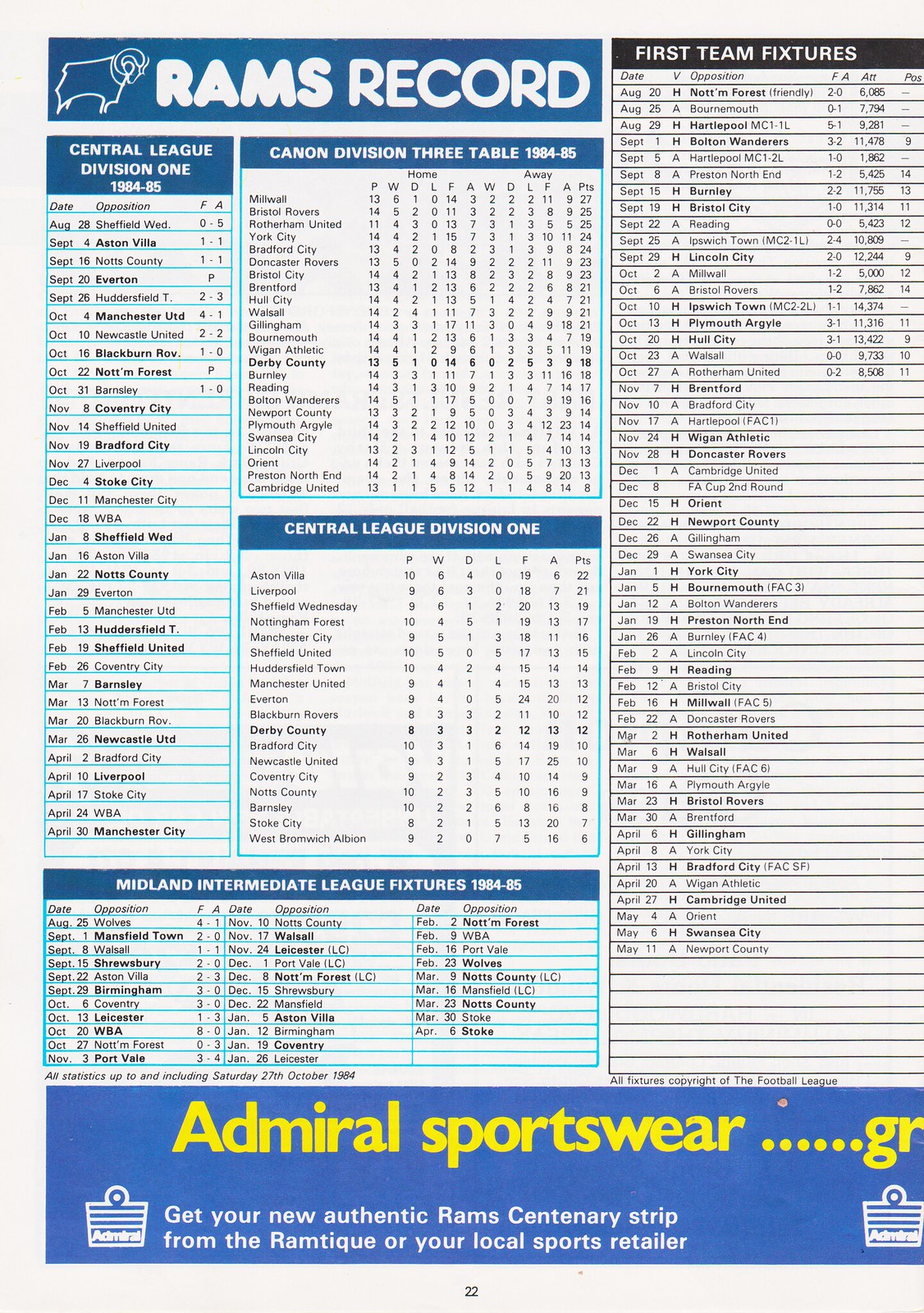The image is a detailed soccer statistics chart with various tables and banners providing comprehensive information on team standings and fixtures for the 1984-85 season. At the very top left, there's a small blue banner with a white silhouette of a ram facing right, accompanied by the text "Ram's Record" in white. Below this banner, the chart is divided into multiple sections.

On the left side, there's a table labeled "Central League Division 1, 1984-85" with rows listing match dates, opposing teams, and scores. Some of the teams mentioned include Sheffield Wednesday, Aston Villa, Notts County, Everton, and Huddersfield Town. To the right of this, another table labeled "Cannon Division 3 Table, 1984-85" shows the standings and game results for other teams.

Further down, there’s a mention of "Midland Intermediate League Fixture, 1984-85," detailing upcoming matches. On the right side of the image, there is a black and white grid titled "First Team Fixtures," listing future games yet to be played.

The entire chart has a white background with prominent teams such as Liverpool, Sheffield, Nottingham Forest, Manchester City, and Everton mentioned multiple times across different divisions. At the bottom of the image, a blue banner with yellow text promotes "Admiral Sportswear," and below that, in white text, there's an advertisement urging readers to "Get Your New Authentic Rams Centenary Strip from the Ramtique or your local sports retailer."